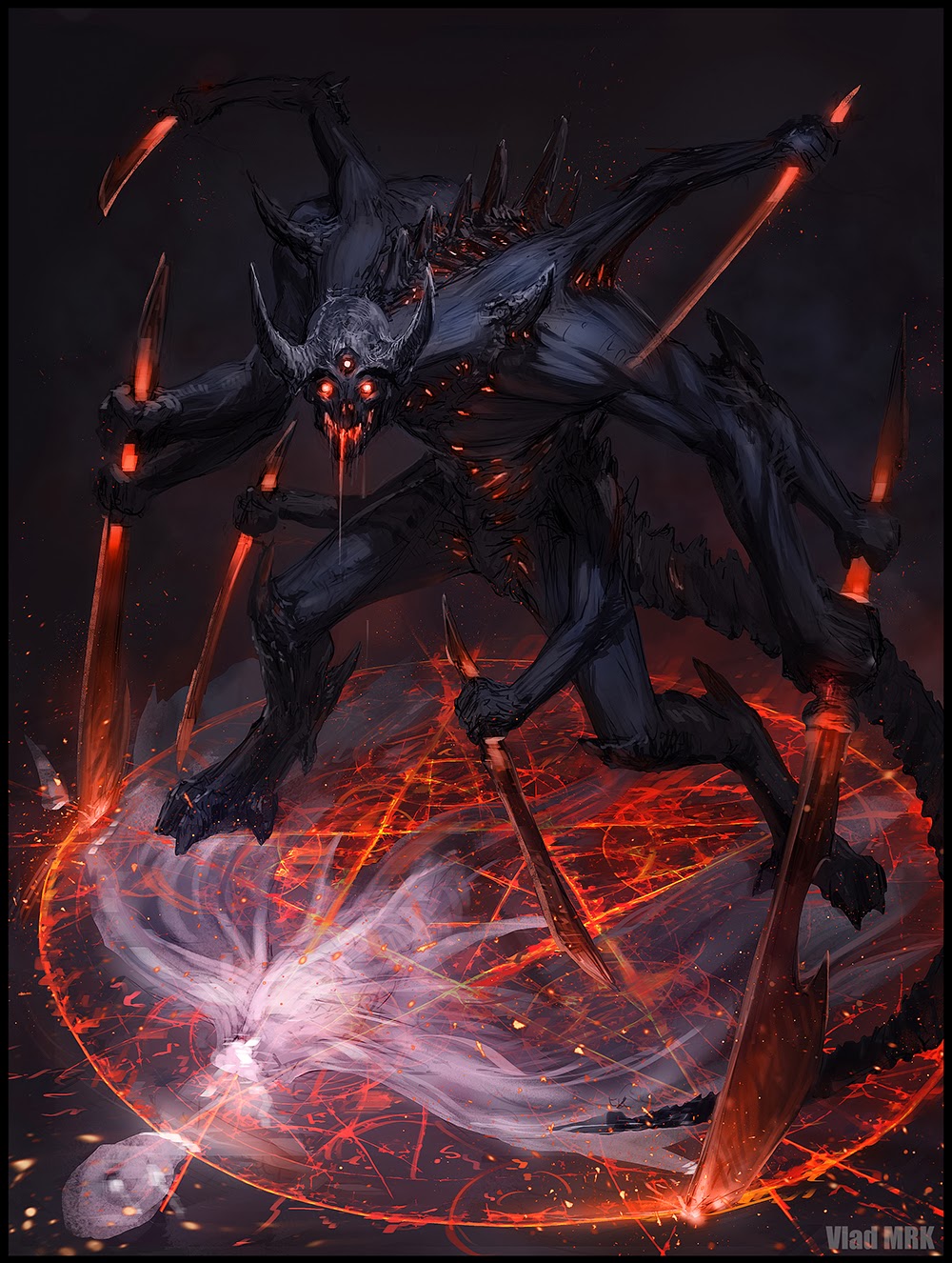The image is a detailed illustration from a fantasy-themed setting, depicting a menacing, black devil-like creature standing in the center of a flaming pentagram. The creature has eight arms, each wielding different flaming swords, and its body is adorned with flames erupting in various places. The monster's form is enhanced with black horns, burning red eyes, a flaming mouth, and spines running down its scaly back, reminiscent of dinosaur legs. Its sinister figure is accentuated by an eerie, oozy red aura. The pentagram itself is fiery red, set against a stark black background and contains the ghostly image of a white figure, perhaps symbolizing an angel, adding to the overall spooky and unsettling effect of the scene.